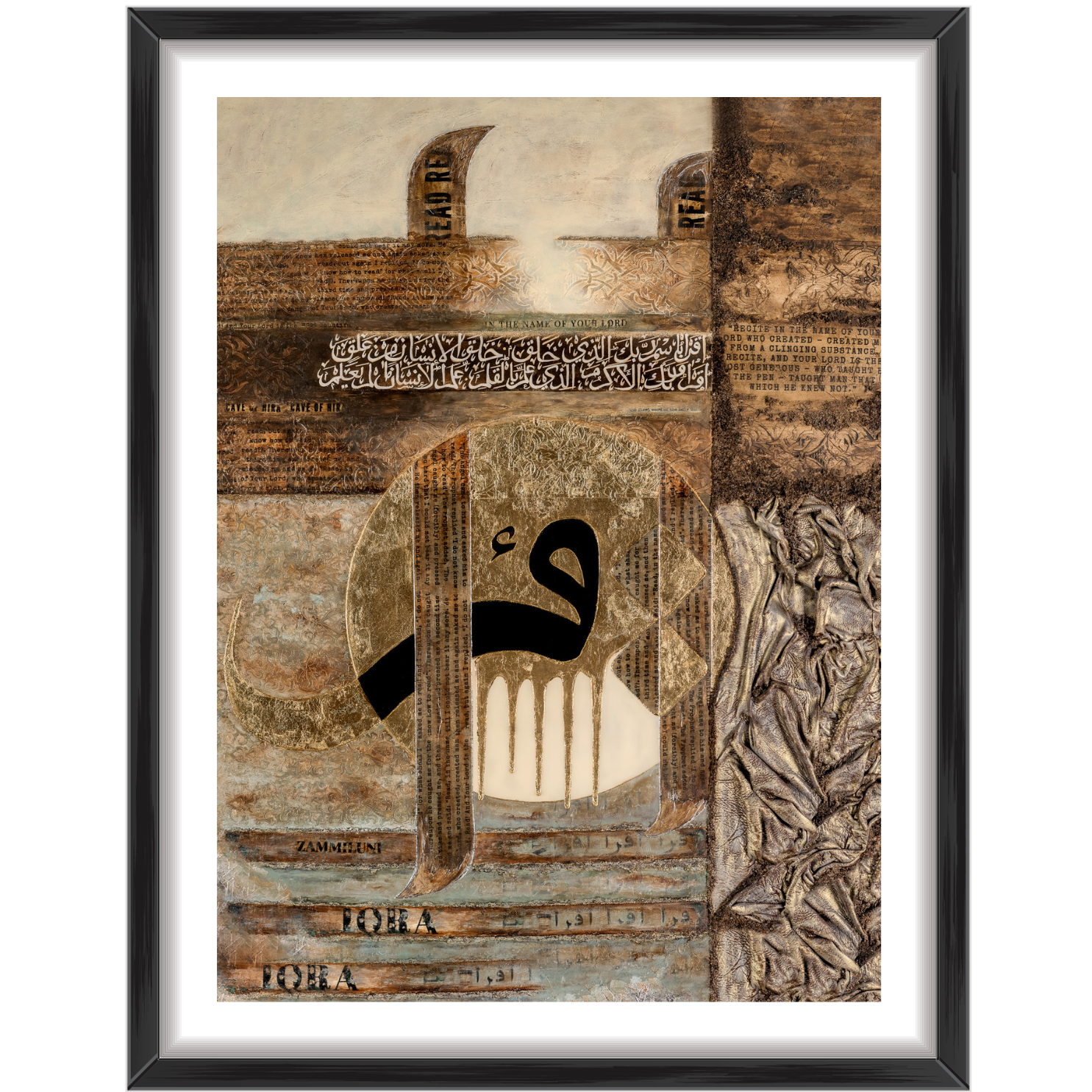This framed artwork is a visually intricate collage composed of antique-looking snippets of Arabic writing and various geometric patterns. The piece is elegantly enclosed within a black frame accented by a white mat, and it is divided into five main sections—two in the upper part, two in the lower part, and a central circular area. Each segment features dominantly inscribed Arabic text, creating an abstract yet harmonious design. The artwork also includes some Latin text in the upper right-hand corner, adding a unique layer to the composition. The textures evoke an old parchment or wall-like surface, enhancing the vintage aesthetic. Rectangular shapes with alternating brown stripes and text populate the bottom portion, adding to the complexity. The right side of the picture includes a lighter brown area, possibly depicting an abstract shape or engraving. In the middle, a large black ribbon traverses the circular central part, with a dripping brown substance adding a dynamic element to the piece.